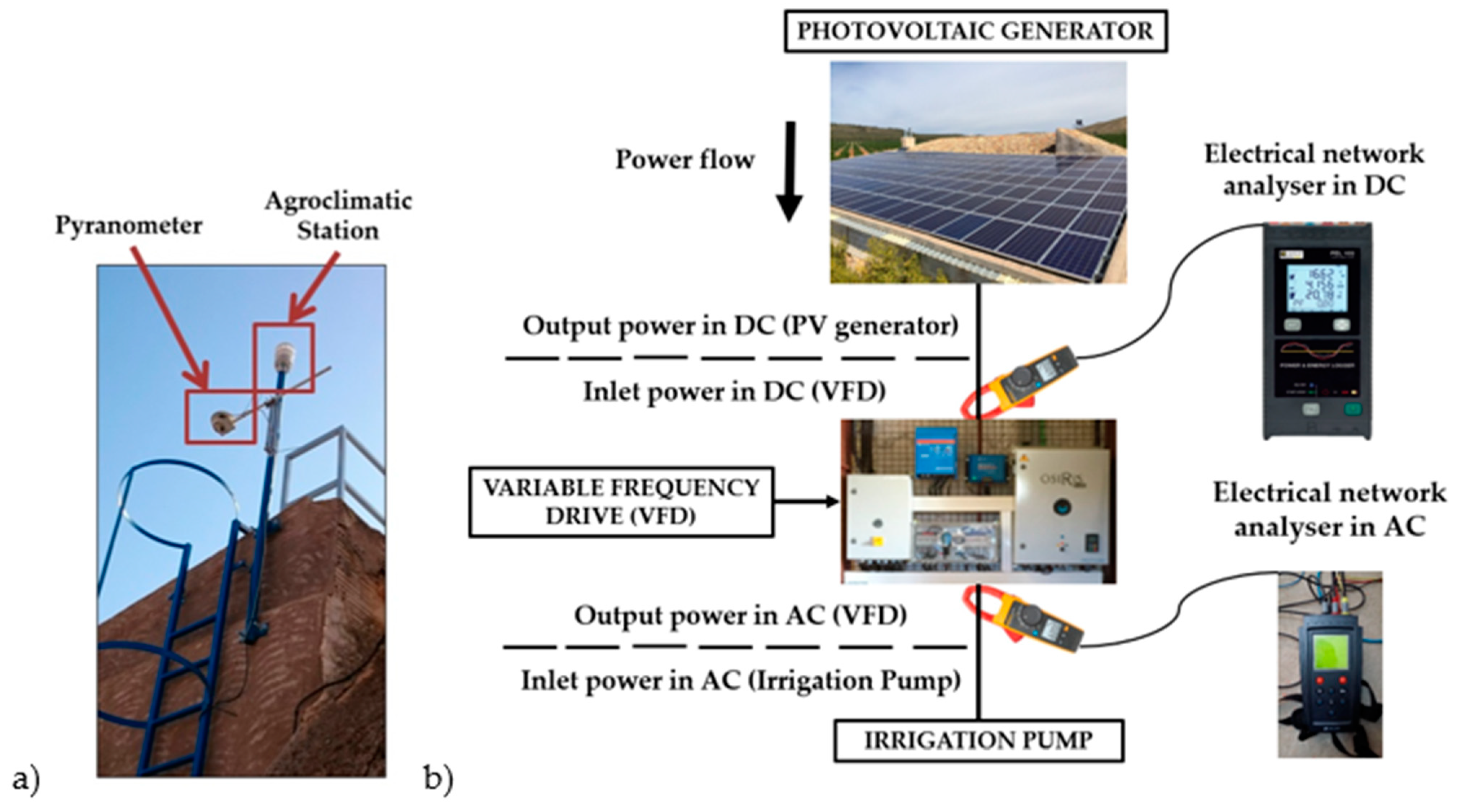This image is a detailed, landscape-oriented diagram illustrating the workings and components of a photovoltaic generator system, with the top and bottom sides being longer than the left and right sides. The diagram is set against a white background and is organized into labeled sections with connecting black lines that explain the relationships between various parts and their functions.

On the left side, labeled as section A, there is a rectangular photograph of an outdoor scene depicting a brick building with an antenna and ladder, identified with red text and arrows pointing to a Pyranometer and Agroclimatic Station. This part focuses on environmental monitoring.

The central section, labeled B, includes two photographs: one of a solar panel at the top and a generator setup in the middle. This section is annotated with black text describing the power flow through the system: "Photovoltaic Generator Power Flow," "Output Power in DC," "Inlet Power in DC," "Variable Frequency Drive," "Output Power in AC," and "Inlet Power in AC."

The right section covers the Electrical Network Analyzers, with two smaller photographs indicating "Electrical Network Analyzer in DC" and "Electrical Network Analyzer in AC."

Throughout the diagram, the text and images are interconnected by black lines, demonstrating the interplay between the various components, culminating in the output to an irrigation pump, illustrating the entire process from energy generation to application.